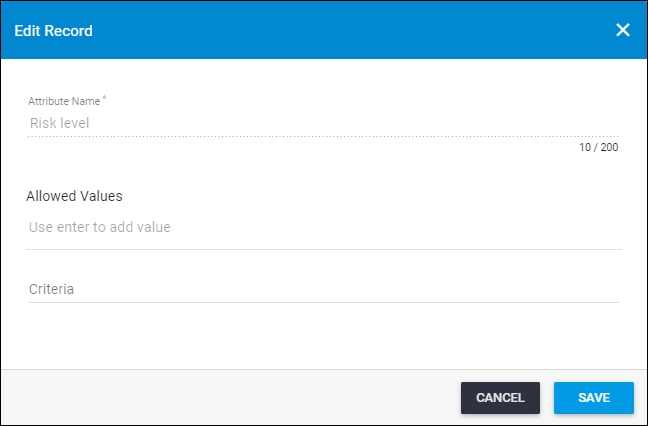The image showcases a compact, pop-up dialog box designed for editing records. The box is bordered with a subtle, black trim. At the top of the box, there's a medium blue banner titled "Edit Record" in a lighter blue font. To the right of the title is an "X" icon, also in a lighter blue hue.

Below the banner is the main section of the box, predominantly white. The first row features the label "Attribute Length Name" in gray text, slightly indented, followed by an editable field labeled "Risk Level." This field currently indicates that 10 out of 200 characters have been used. 

Further down, in bold black text, the phrase "Allows Loud Values" appears, also indented, with a blank field below it labeled "Use Enter to Add Value," suggesting an input limit on characters as well. 

Below this, there is another input field, slightly darker in gray, labeled "Criteria," allowing users to type in their criteria.

At the bottom of the dialog box, there is a gray banner with two buttons on the right side: a black "Cancel" button and a blue "Save" button, both ready for user interaction.